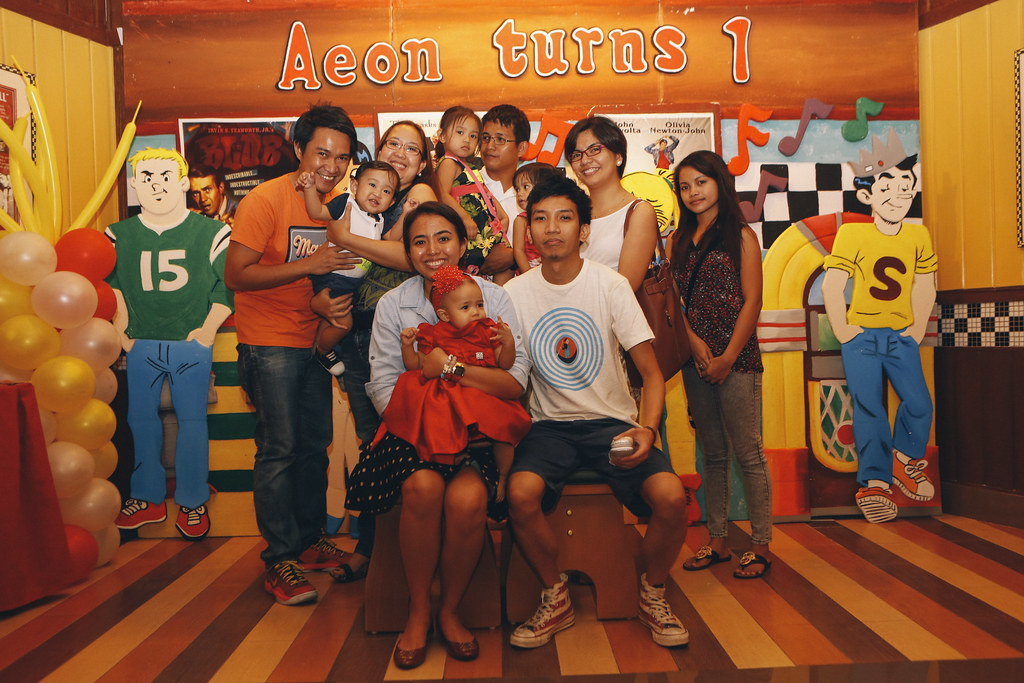This vibrant image captures a joyous family celebration, most likely a baby girl's first birthday, as suggested by the cartoon-style text at the top that reads "Aeon Turns One." The venue is decorated in a fun and colorful theme, reminiscent of an entertainment or play area, featuring iconic Archie characters. To the left of the gathering, there's a cardboard cut-out of Jughead standing in front of a jukebox, next to a tall tower of yellow, white, and red balloons. The entire room is decorated in a lively orange and yellow color scheme, with the wooden floor sporting stripes of brown, orange, and yellow.

Central to the image is the family, showcasing a mix of adults, teenagers, and children, all dressed in various colors such as white, blue, orange, and red. In the front, a young couple in their 20s sits on a bench, proudly holding a baby girl in a red dress, presumably Aeon. Behind them are more family members, including two other couples each holding young children—a two-year-old boy and a two-to-three-year-old girl—indicating a multi-generational gathering. Everyone appears to be in high spirits, contributing to the festive atmosphere of this memorable celebration.